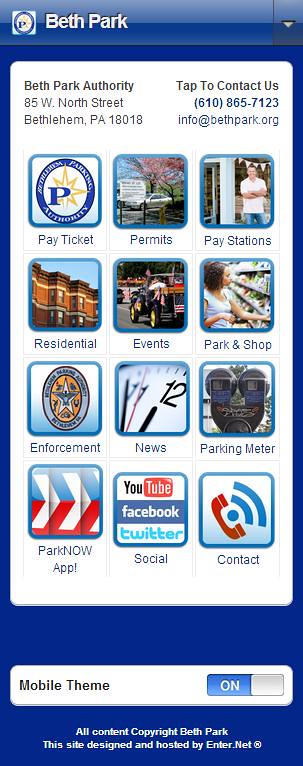The photograph captures what appears to be an enlarged screenshot of a cell phone displaying a detailed information sign for Beth Park. At the top, in white letters on a blue background, it reads "Beth Park." Below, in a rounded rectangular section with a white background, it states "Beth Park Authority," along with the address "85 West North Street, Bethlehem, PA 18018" and a contact prompt "tap to contact us," followed by the phone number "610-865-7123" and the email "info@bethpark.org." The middle section features four rows and three columns of interactive buttons labeled with icons. The first row includes "pay ticket," "permits," and "pay stations," followed by "residential," "events," and "park and shop" in the second row. The third row lists "enforcement," "news," and "parking meter," while the final row shows "park now app," "social," and "contact.” At the bottom of the screen, it notes "mobile theme on" in a white rectangular area, with a final blue strip stating "all content, copyright Beth Park," and the website design and hosting credited to "inter.net."